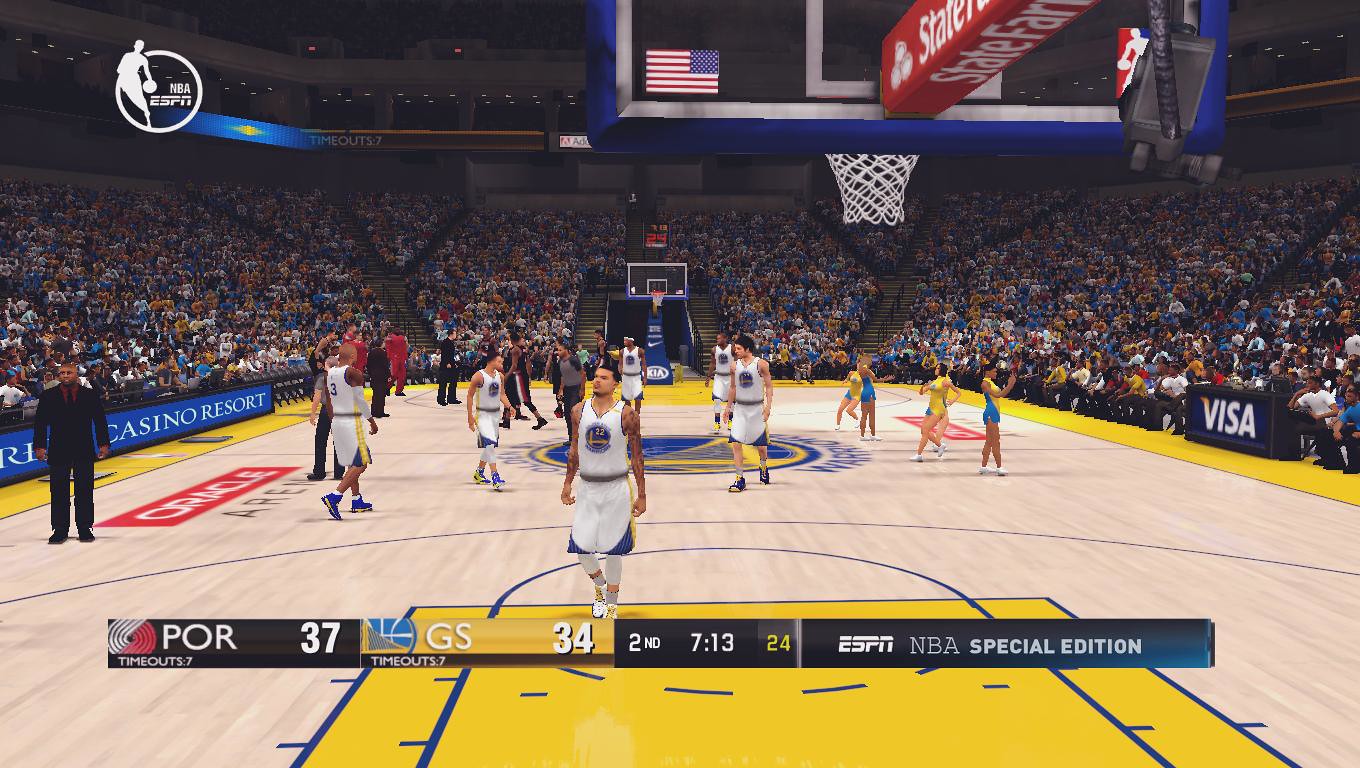This wide-angle photograph captures the intensity of a basketball game happening on an indoor court, framed from just below the net at one end and extending across to the furthest basketball backboard at the other end. The stadium is packed with spectators, giving the scene a lively and crowded atmosphere. The focus of the players is toward the center of the court, actively engaged in the game, while cheerleaders can be seen on the right side, facing the enthusiastic crowd. A prominent black banner marked 'VISA' is positioned between the cheerleaders and the audience on the right. The left side of the image features a blue banner, partially obscured, with a man in black attire standing in front of it, likely a coach or official. 

The upper left corner of the image includes the recognizable NBA logo, alongside ESPN branding, indicative of the game's significant coverage. The bottom section of the photograph overlays a detailed score banner: 'POR 37' signifying the Portland Trail Blazers leading with 37 points, next to 'GS 34' representing the Golden State Warriors with 34 points. Additional details such as '2ND 7:13', representing the second quarter with 7 minutes and 13 seconds remaining, '24', likely the shot clock, and 'ESPN NBA Special Edition' enhance the informative and immersive presentation. Additional elements include the Golden State Warriors logo on the court and a State Farm logo at the top goal, emphasizing that the game is held on Golden State's home ground. The crowd and perhaps some elements on the court appear virtually generated, adding a unique twist to this dynamic sports scene.